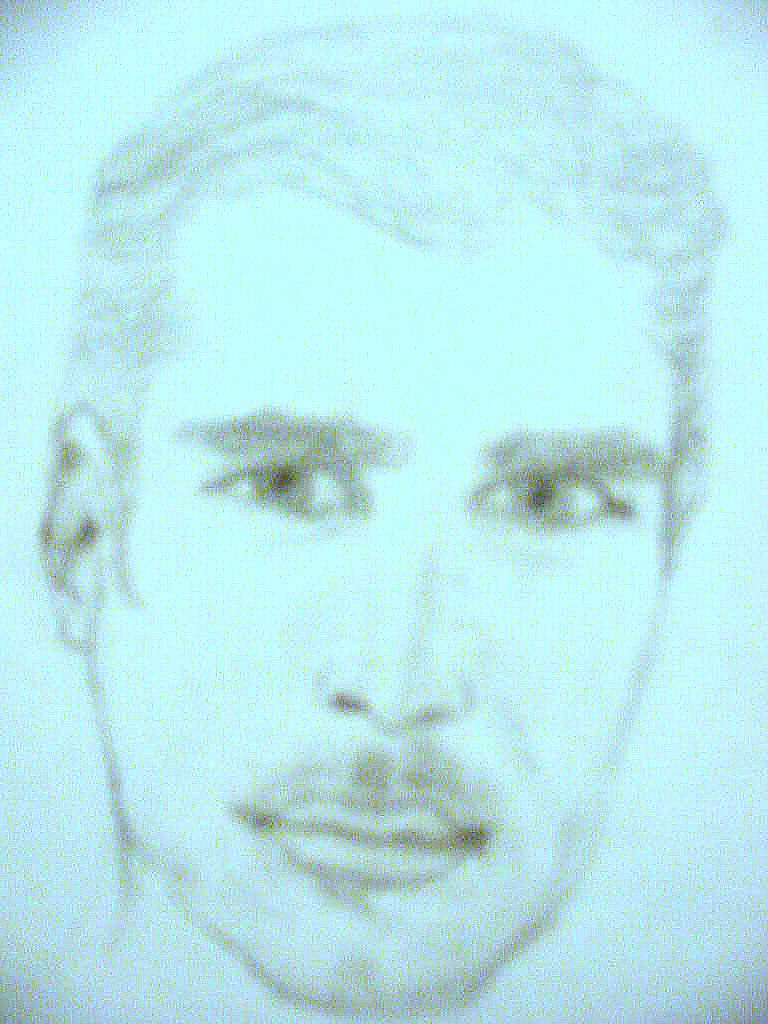This portrait drawing of a man, executed in blue with black pencil accents, has a grainy texture that intensifies towards the bottom. The subject's wavy hair, relatively long at the top, appears slicked back behind his ears. His bushy, lowered eyebrows frame light-colored eyes that sit evenly across his face. A sharp, slightly wide nose leads down to his full lips, which are partly obscured by a subtle mustache. The drawing also reveals part of his ear and a portion of his neck, with a distinct cleft in his chin adding character to his visage.